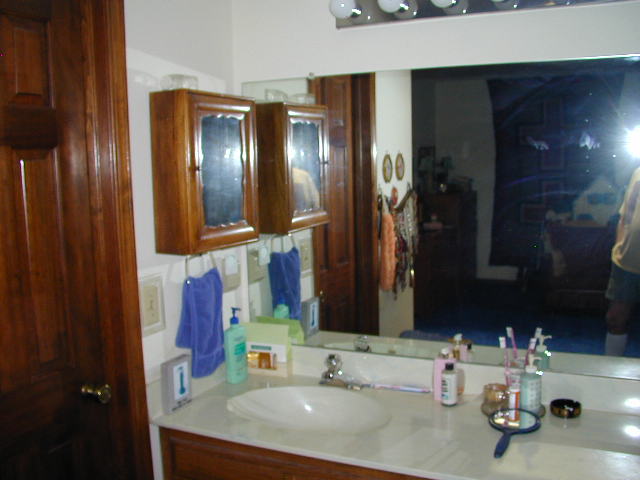The photograph depicts a bathroom, captured with a flash. The centerpiece of the image is a long bathroom vanity, positioned beneath a large mirror that reflects a portion of an adjacent room. The flash creates a bright reflection on the right-hand side of the mirror, suggesting an open door and revealing a glimpse into another room, possibly a bedroom or living room, where a chair is visible.

The vanity itself is notably long but houses only a single sink located on the left side, which contrasts with the empty counter space on the right. The sink is oval-shaped, featuring a silver-toned faucet, likely made from Corian or a similar material. Above the vanity, a brown wooden cabinet with a mirror is mounted on the wall, with a medium blue towel hanging from a handle below it.

The countertop is relatively uncluttered, with a few personal items scattered across its surface. On the left side, there's a green pump bottle of lotion and an indistinguishable object behind it. To the right of the sink, a toothbrush lies on its side alongside a pink bottle and a white bottle containing some liquid. A dark blue hand mirror, a toothbrush holder with a couple of toothbrushes, and possibly an ashtray are also present. The vanity's cabinetry features somewhat dark brown wood, visible in the doors and the trim beneath the countertop.